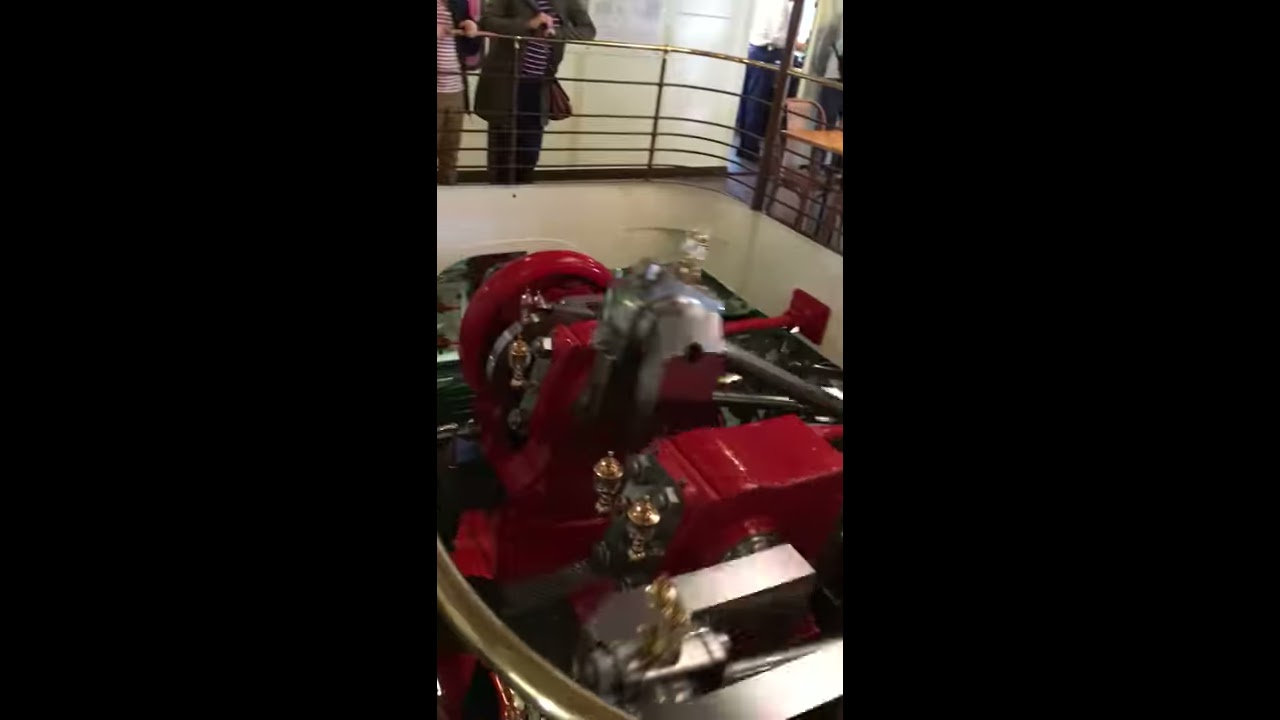This photograph captures a detailed scene of an enigmatic, vibrant red mechanical contraption, possibly an antique engine or an old-fashioned car, adorned with gold and brass components that evoke a vintage aesthetic. The intricate machine is set within a fenced-in area amidst a beige room, illuminated by natural daylight streaming through windows in the background. The setting resembles a museum or a display area with scattered tables and chairs, hinting at a restaurant-like environment.

Two individuals are leaning over a gold railing, closely inspecting the contraption. The first person, whose top half is visible, wears an olive-colored jacket over a purple and white striped shirt paired with black pants. The second individual, glimpsed from the waist down, sports a pink and white striped shirt with dark khaki trousers. Their absorbed attention towards the mechanical piece, combined with the absence of explanatory text or signage, suggests an exhibit designed to intrigue and invite speculation about its purpose and history.